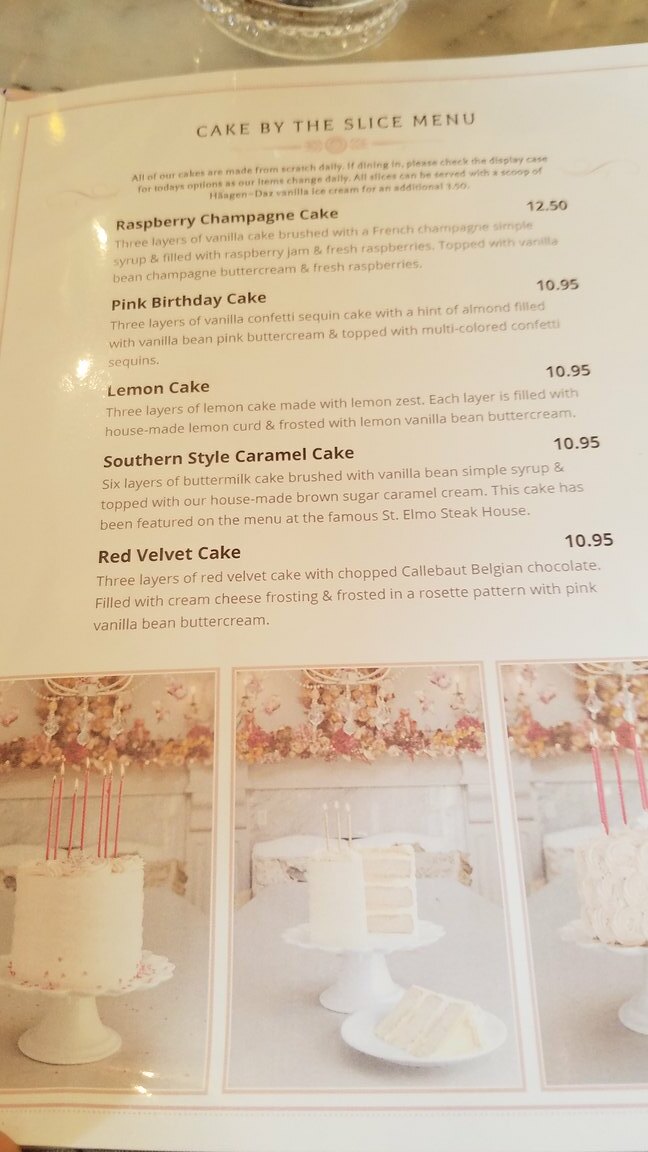This image features a photograph of a menu labeled "Cake by the Slice Menu," captured with a standard camera. The top section of the menu includes a brief paragraph, although its text is too small to decipher clearly. Below the introductory text, a variety of cakes are listed with prices and descriptions:

1. **Raspberry Champagne Cake** - Priced at $12.50, accompanied by a faint and difficult-to-read description.
2. **Pink Birthday Cake** - Priced at $10.95.
3. **Lemon Cake** - Priced at $10.95.
4. **Southern Style Caramel Cake** - Priced at $10.95.
5. **Red Velvet Cake** - Priced at $10.95.

Each cake name is prominently bolded in black for easy reading, with more descriptive paragraphs in a rosy hue underneath each listing, explaining the ingredients and details about the cakes. 

At the bottom of the menu, there are three photographs of different cakes. The central image showcases a cake cut in half, revealing its three-layer structure. The cakes on either side are adorned with long, pink candles.